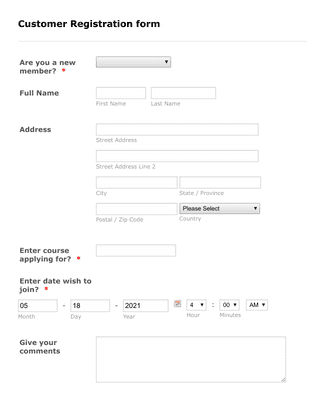The image depicts a web page dedicated entirely to a customer registration form set against a clean, white background without any borders. At the very top of the page, bold black text declares "Customer Registration Form." Directly below this title, a very pale, thin gray line extends across the screen, delineating the header from the form itself.

Below this line, on the left-hand side, bold gray text asks "Are You a New Member?" followed by a red asterisk indicating a required field. To the right of this question is a gray dropdown box. The subsequent section of the form, labeled in bold text, reads "Full Name," accompanied by two white boxes with light gray borders for entering the first and last names, respectively. 

Further down, bold text prompts the user to fill in their "Address," with designated white boxes for street address, street address line 2, city, state/province, and zip code. Adjacent to the zip code field, there is a gray dropdown box with the placeholder text "Please Select" and beneath it, in smaller light gray text, the word "Country." Additional white boxes for country input follow below this section.

Continuing the form, the next section instructs users to "Enter Course Applying For," marked with a red asterisk, in bold text. Following this, another bold text instruction reads "Enter Date, Wish to Join," also with a red asterisk. The relevant fields for this section are already filled with the value "6-18-2021." To the right of these date input boxes are additional fields to specify the hour and minute, which are populated with "4 AM."

At the bottom of this form, there is a larger text box, outlined in light gray, designated for comments, labeled "Give Your Comments." This box is currently empty. The entire layout is both functional and visually clear, with a consistent use of gray and white tones and selective bolding to guide the user through the registration process effectively.